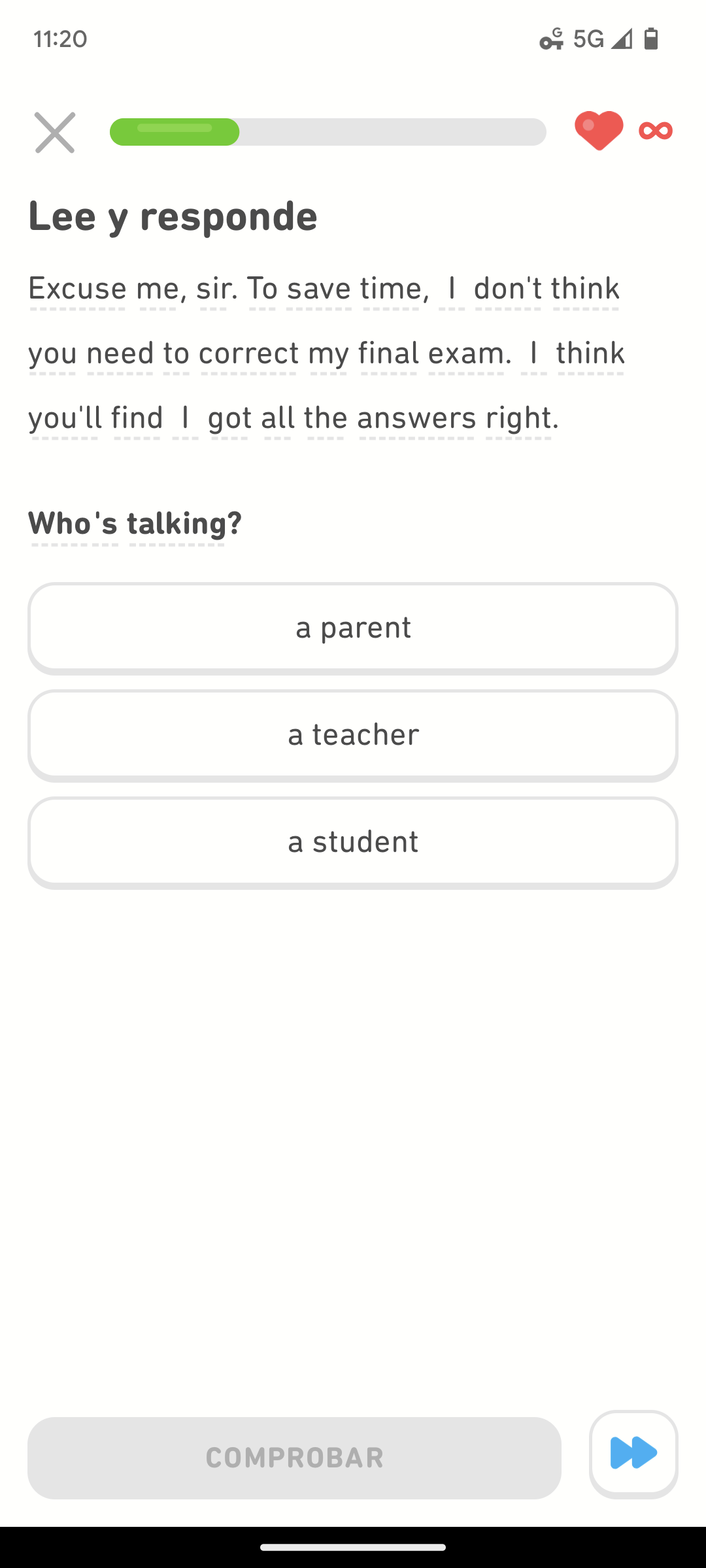Caption: 

A detailed screenshot of a test prep application is displayed. In the top left corner of the interface, a large "X" icon allows users to exit the current question. At the center of the screen, a progress bar indicates the user's advancement, showing that only a quarter of the test has been completed. The progress bar is partly filled with green, reflecting the minimal progress made so far. To the right of the progress bar, heart and infinity sign icons are both highlighted in red, suggesting they have been selected.

Below the progress bar, on the left side, some introductory text is partially visible. Moving further down, a message indicates user confidence by stating: "I think you'll find I got all the answers right." Directly below this message are three vertical boxes listing different possible answer choices: "a parent" at the top, "a teacher" in the middle, and "a student" at the bottom.

Towards the bottom left of the screenshot, a large gray section is present. Accompanying this section on the right is a white box containing two blue arrows, both pointing to the left, perhaps representing navigation controls.